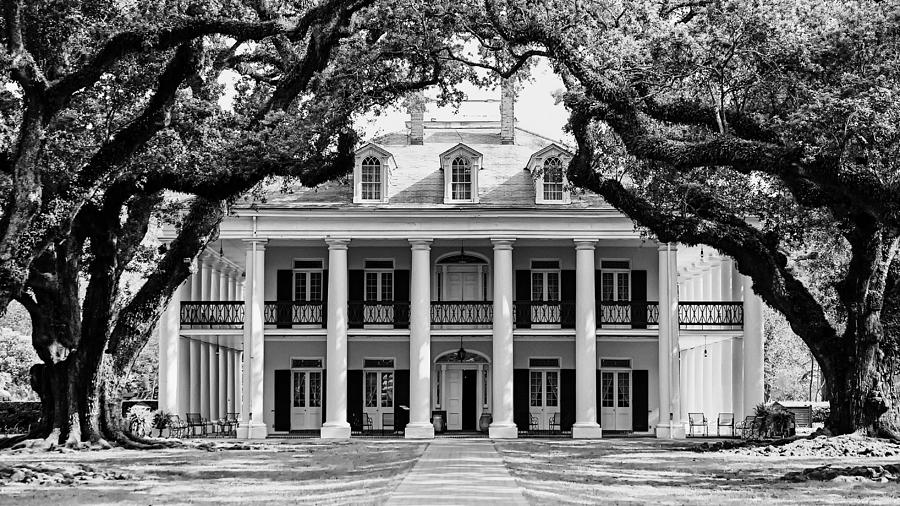This black and white photograph captures a grand, stately mansion from a front perspective. The mansion is likely light-colored, with darker accents surrounding the door and window frames. A central pathway leads directly to the entrance, which features double doors, one of which is open. An identical set of double doors on the second level opens onto a balcony that extends around the entire house. The mansion is supported by eight stately stone columns, which uphold an angled roof with three prominent dormer windows, likely indicating an attic space. The house is framed on either side by two large, mature trees, possibly oaks, whose branches arch overhead and converge, partially covering the house. The left side of the mansion features some seating, akin to a patio, adding a homely touch to the grandeur. Overall, this elegant estate exudes an old-fashioned, possibly governmental or manorial charm, underscored by its expansive design and stately architectural features.